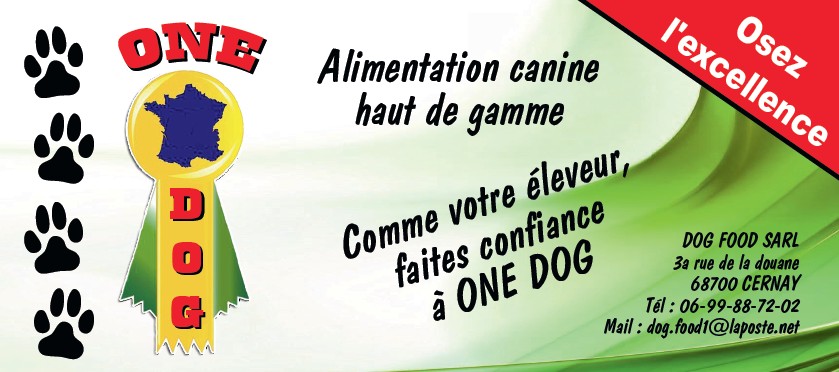The image depicts a computer-generated banner for a high-end dog competition or dog show. It features a series of four black dog paw prints arranged vertically on the left side against a white background. Central to the image, a colorful logo with the text "One Dog" prominently displays, with "One" in large red letters above a yellow medal with a ribbon where "dog" is written in red text. Green waves adorn the background on the right side. To the right of the logo, text in French reads "Alimentation Canine Haute de Gamme" and "Comme Votre Éleveur, Faites Confiance à One Dog", emphasizing its premium dog food. The upper right corner includes a red triangle with white lettering that says "Osez l'Excellence", and the bottom right corner against a green backdrop provides contact information: "Dog Food S-A-R-L, 3A Rue de la Douane, 68700 Cernay", along with a telephone number "06-99-88-72-02" and an email address "dog.food1@laposte.net".